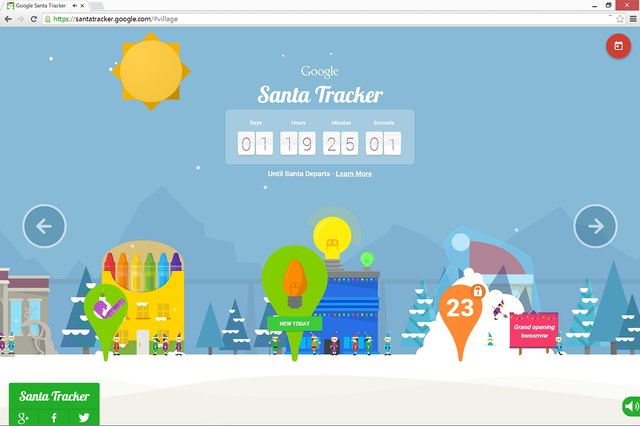The image depicts the Google Santa Tracker website. At the top-left corner of the browser tab, "Google Santa Tracker" is indicated, and on the top-right, the typical browser control buttons — a red background "X" for close, a double square for minimizing/maximizing, and a minus symbol for minimizing — are present. The URL bar shows the secure HTTPS designation in green text, followed by the web address: santatracker.google.com/#village.

In the center of the webpage, the title "Google Santa Tracker" is prominently displayed. Below the title, a countdown timer is shown, segmented into days, hours, minutes, and seconds. The current countdown reads: 01 day, 19 hours, 25 minutes, and 01 second.

In the top-left section of the website, a bright yellow sun illuminates the scene. The bottom half of the screen showcases a whimsical village landscape. Highlights include a blue building with a yellow light atop it. Additionally, to the left of this structure, there's an artistic storage resembling crayons, lined up in red, orange, yellow, green, blue, and purple, evoking a colorful and playful atmosphere.